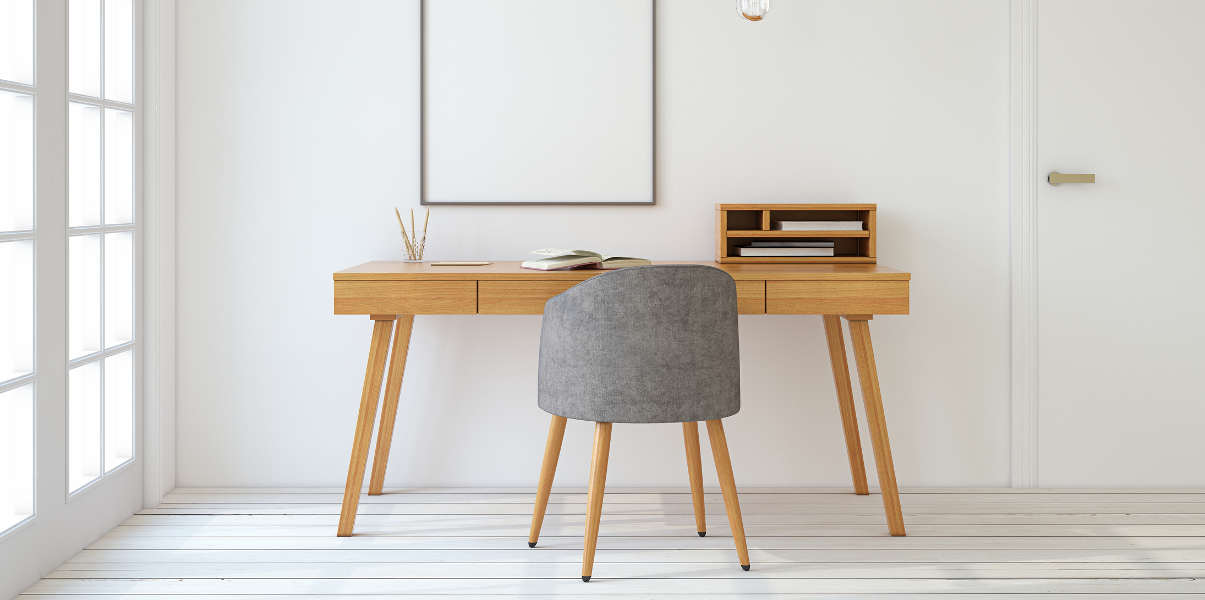The photograph captures a bright, minimalistic office room bathed in natural, white light. On the left, large French doors with glass panes allow daylight to flood in, illuminating the white walls and enhancing the room's airy aesthetic. Adjacent to these doors is a spacious window, its frame featuring white slits. Dominating the center of the room is a sleek, light brown wooden desk positioned beneath a whiteboard with a thin black frame. The desk is meticulously organized, with an open book in the middle, a pen holder to the left, and additional stationery. In front of the desk stands a low-backed gray chair with matching wooden legs. To the right of the desk, there's a two-tier wooden cubby filled with books and papers. Beyond this, a white door with a gold handle provides access to the room. The white carpeted floor with subtle horizontal pinstripes completes the pristine look of this home office.